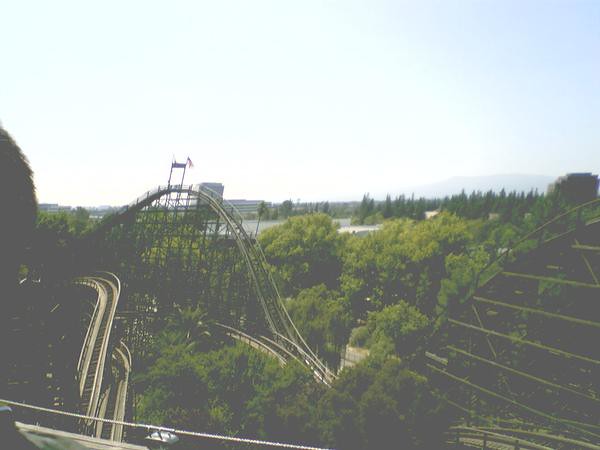This aerial photograph showcases a wooden roller coaster nestled within a lush landscape of fully grown green trees under a smooth, bluish-gray sky. The image, slightly fuzzy and taken in bright sunlight, reveals a roller coaster track emerging from the dense foliage. The track ascends into a high hump at the left of center, adorned with a giant gate and two flags at its peak, before dramatically dipping and rising into another hill at the image’s edge. To the left, another section of track, possibly from a different ride, suggests a complex amusement park setup. Despite the fog-obscured hill in the background, the vibrant greenery and the towering roller coaster structure dominate the scene, evoking the lively essence of a summer day adventure.